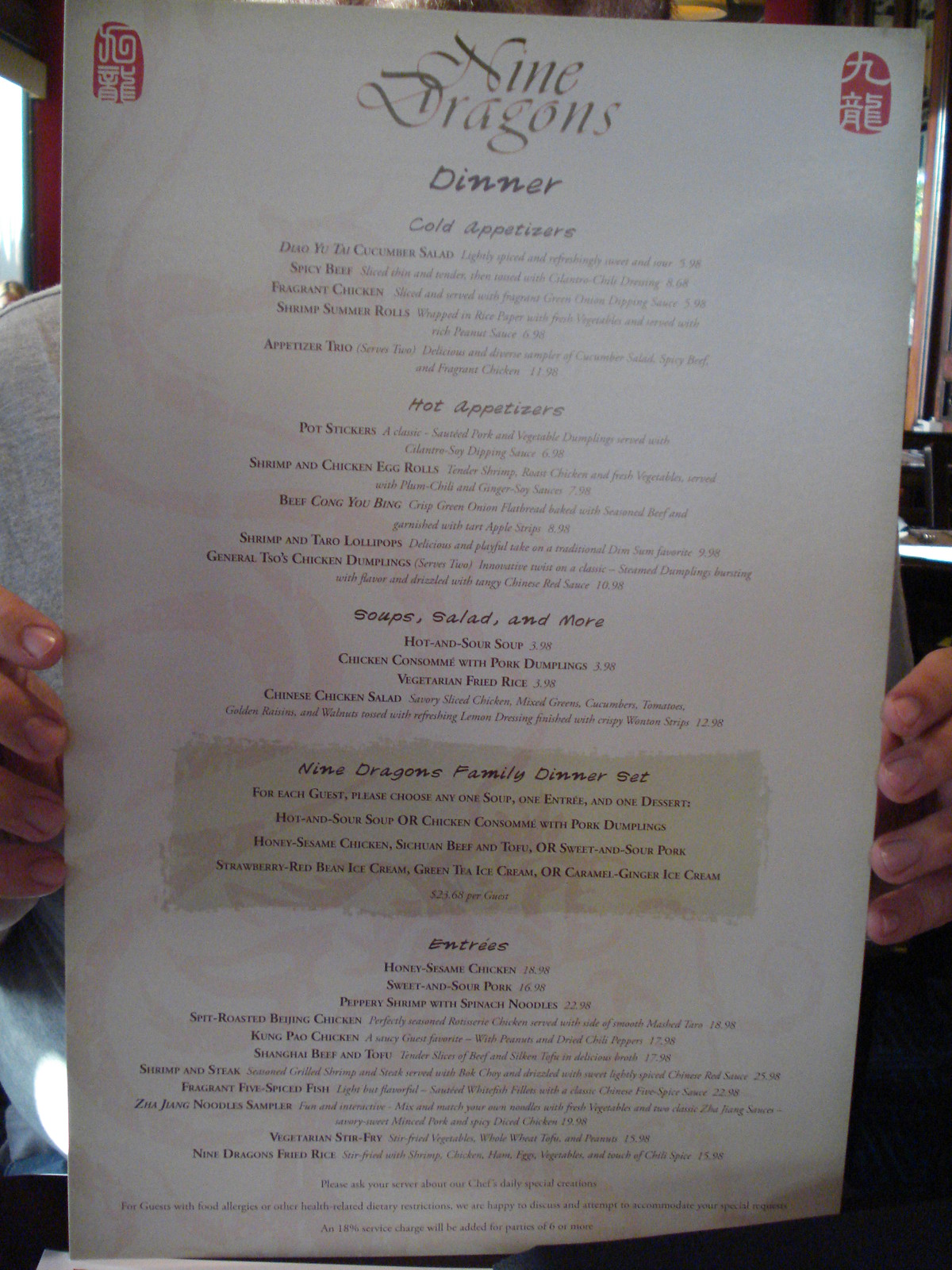This image depicts a detailed menu from the Nine Dragons restaurant. The menu begins with a selection of cold appetizers, featuring items such as cucumber salad, spicy beef, fragrant chicken, and shrimp summer rolls. There is also an appetizer trio option available. 

Moving on to hot appetizers, diners can choose from potstickers, shrimp and chicken egg rolls, beef Kong Yo Bing, and shrimp and taro lollipops. The menu highlights a special item: General Tso's Chicken Dumplings, which sounds particularly appetizing.

The soups section offers a variety of choices, including hot and sour soup, chicken consommé with pork dumplings, and a vegetarian option. For those seeking rice dishes, vegetarian fried rice is available. Additionally, the menu lists a Chinese chicken salad.

For a more comprehensive dining experience, the Nine Dragons family dinner set includes one soup, one entrée, and one dessert, providing a well-rounded meal option. Overall, the menu offers a diverse array of flavorful and intriguing dishes.